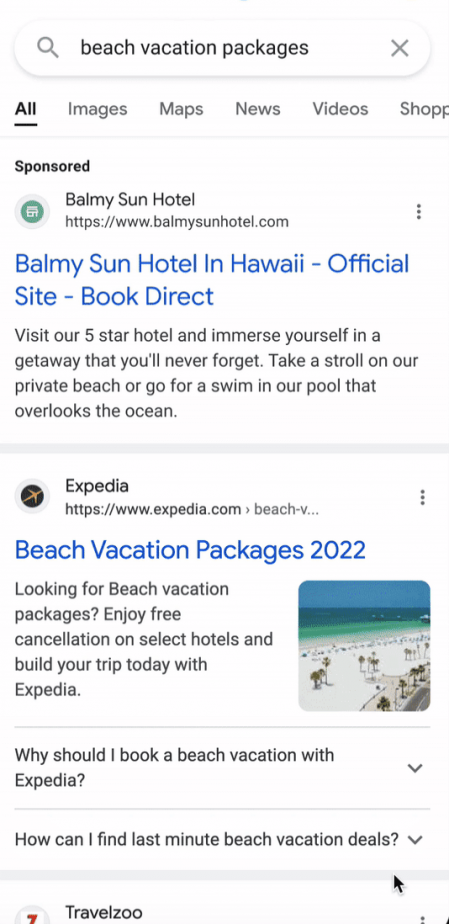The image depicts the interface of a search engine, possibly Google or Bing, with the search query "Beach Vacation Packages" entered in the search bar. The search bar features a magnifying glass icon on the left and an X icon on the right. Just below the search bar, a horizontal menu displays categories including All, Images, Maps, News, Videos, and Shopping, with the "All" category currently selected, indicated by bolded black text and a black underline.

Underneath this menu, there is a section labeled "Sponsored" in bold black text, followed by a sponsored listing for the Balmy Sun Hotel. The link for the hotel is www.balmysunhotel.com. Its description reads, "Visit our 5-star hotel and immerse yourself in a getaway that you'll never forget. Take a stroll on our private beach or go for a swim in our pool that overlooks the ocean."

The second link provided is for Expedia (www.expedia.com), with the title "Beach Vacation Packages 2022." Below this link are two expandable sections labeled "Why should I book a vacation with Expedia?" and "How can I find last-minute beach vacation deals?" each featuring a downward arrow to the right, indicating that further information can be viewed.